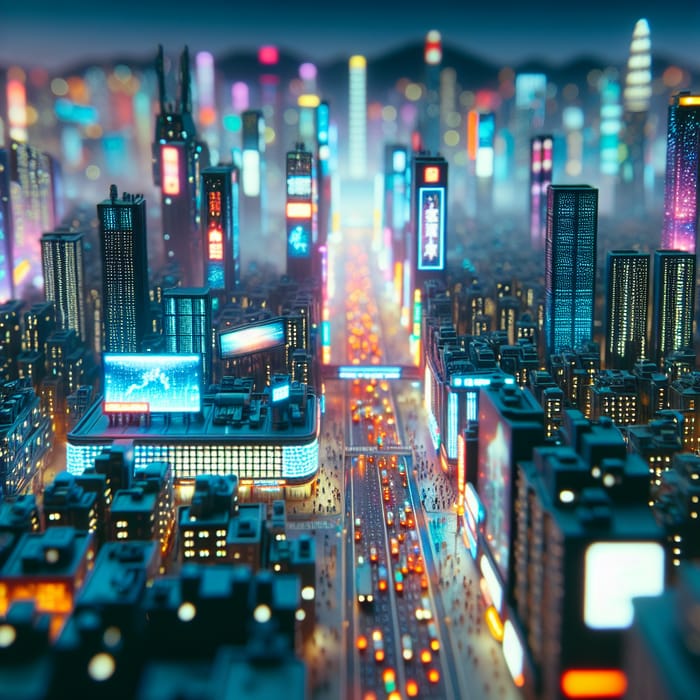This digitally enhanced, stylized night scene captures a sprawling urban landscape reminiscent of Tokyo or a similarly vibrant city. The centerpiece of the image is a major roadway, splitting the composition from bottom to top, bustling with an array of vehicles including cars, trucks, and buses. The roadway, consisting of eight lanes, is portrayed in sharp relief at the foreground and gradually fades into the distance, giving the impression of depth.

Flanking this main drag are towering skyscrapers and tall buildings adorned with countless neon signs and billboards, their brightly colored lights punctuating the largely shadowed cityscape. The foreground buildings, with illuminated office windows, are darker and more defined, while those receding into the background appear blurrier and more vibrant, creating a distinctive dotted effect against the night sky.

The vehicles, which look like smooth, toy-like cars, are depicted with their headlights facing the viewer on the left side of the road and tail lights on the right, indicating the flow of traffic in both directions. The city's skyline, dotted with brilliantly colored structures in hues of bright light blue, purple, and red, is set against the backdrop of a dark mountainous ridge and a deep blue night sky, contributing to an artistic and somewhat surreal atmosphere.